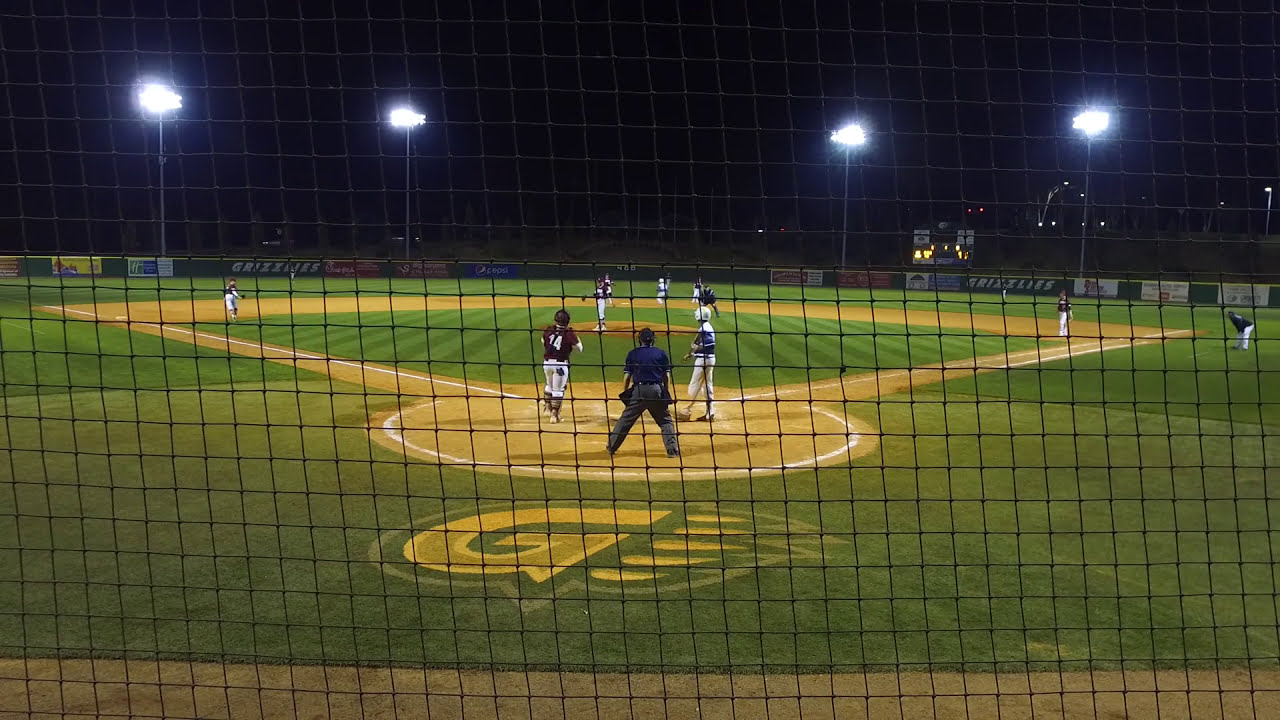This nighttime baseball game photo, shot from behind home plate, captures a dynamic scene under a pitch-black sky illuminated by towering, bright stadium lights. The green field is clearly visible with the baseball diamond laid out in front. The view is through protective netting directly behind the umpire, who is clad in gray pants and a blue shirt. In the frame, the batter stands poised with a blue top and white pants, while the catcher in a red top marked with the number 14 appears ready to throw the ball back to the pitcher. Surrounding the field are logos and signs, including a prominent yellow 'G' adorned with flames or wings. The shot encompasses first base to the right, third base to the left, and second base off in the distance, showcasing the full layout of the field and adding to the context of this immersive night game moment.